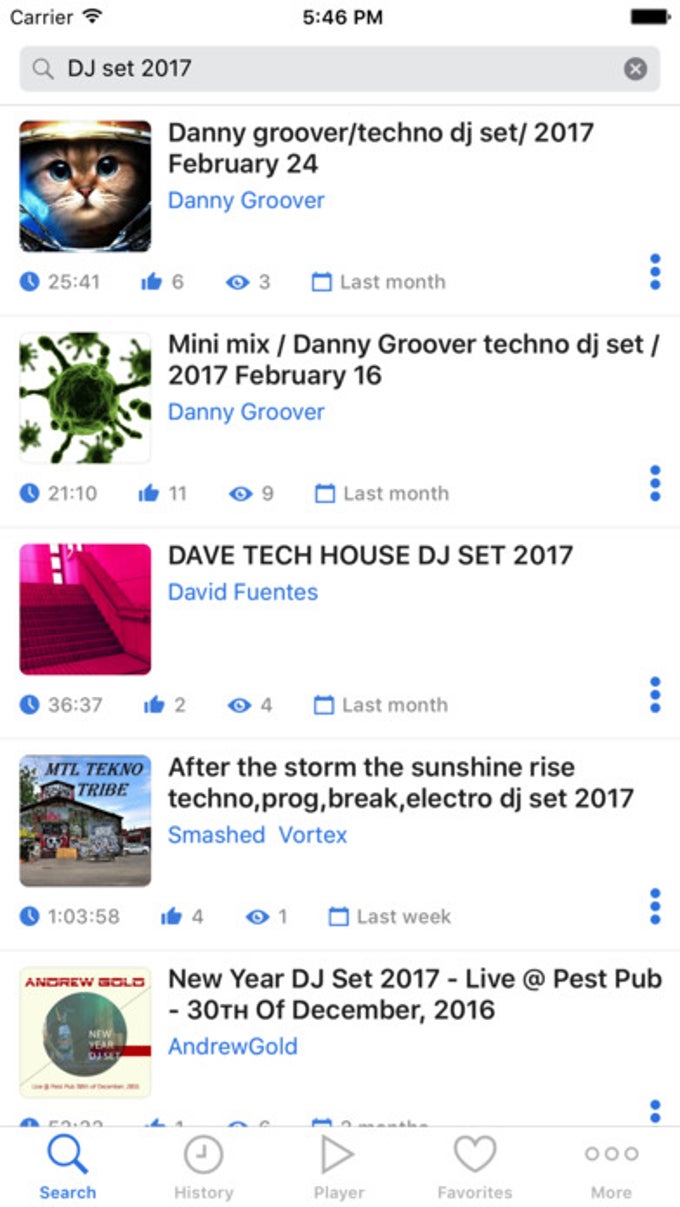This is a detailed screenshot from a smartphone displaying the interface of a music streaming app, resembling Spotify. The image clearly indicates it is a mobile screenshot as evidenced by the phone's status bar at the top, showing the remaining battery life, current time, Wi-Fi signal strength, and the carrier's name. At the bottom, typical phone menu icons are partially visible. The main content reveals search results for the term "DJ set 2017." 

Several playlists and DJ sets are shown, each accompanied by a small icon, which varies from digital artwork to non-photographic designs. Prominent entries include "Danny Groover Techno DJ Sets," "Mini Mix," "Dave Tech House DJ Sets," "New Year DJ Set 2017," "After The Storm," and "The Sun Shine Rise Techno." Each entry displays supplementary information such as duration, the number of likes, the count of listeners, and the upload date, providing a comprehensive overview for the user.